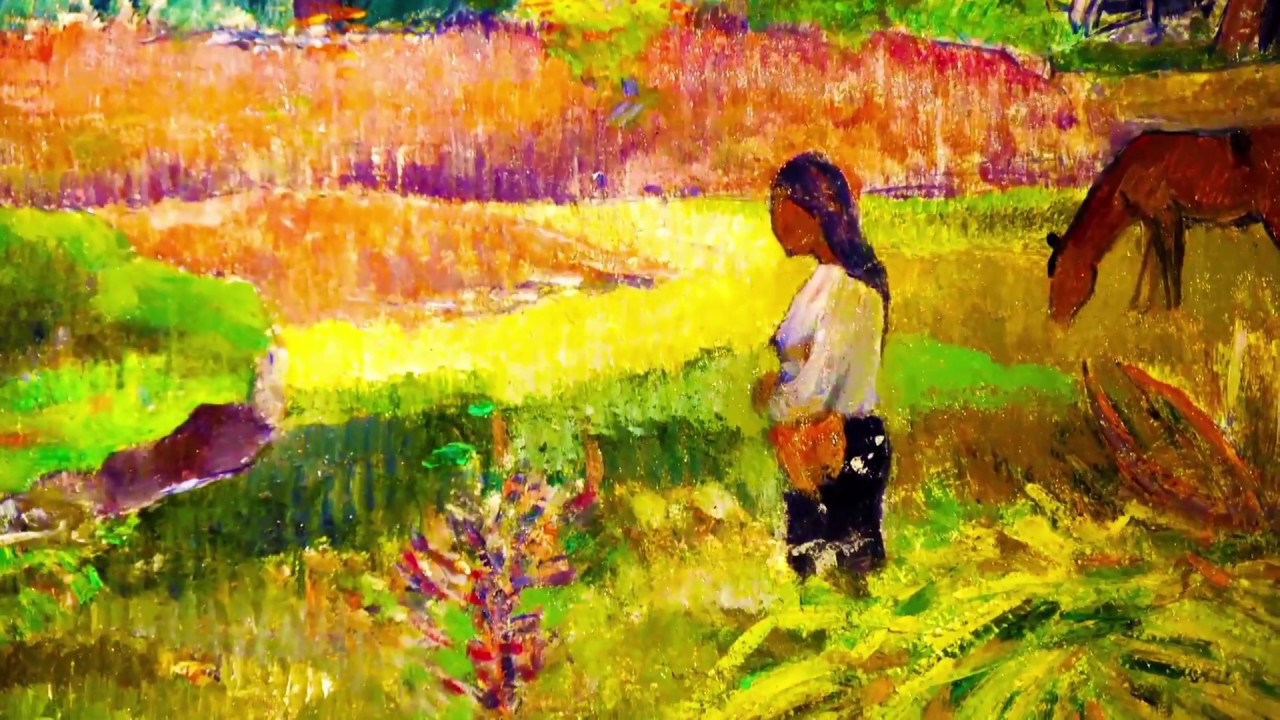The image is a vividly colored painting, rendered in thick, dense brushstrokes that hint at the use of pastels or oil pastels. Central to the composition, just off-center, is a medium dark-skinned woman with long, black hair. She is adorned in a white top and black pants and holds an orange object which could be a bag. The woman lacks defined facial features and faces left, standing knee-high in a vibrant field of yellows, greens, and browns. In the background, to the right, a faceless brown horse is grazing, while on the left, a bird (or possibly a turkey) catches her gaze. The abstract background teems with lively hues of green, orange, yellow, purple, and pink, with patches of red and peachy orange in the upper section, suggesting a wild, lush landscape under a colorful sky speckled with shades of blue, white, dark green, and lime green. The overall ambiance and style suggest the work of a possibly inexperienced native painter, potentially hailing from Central America.